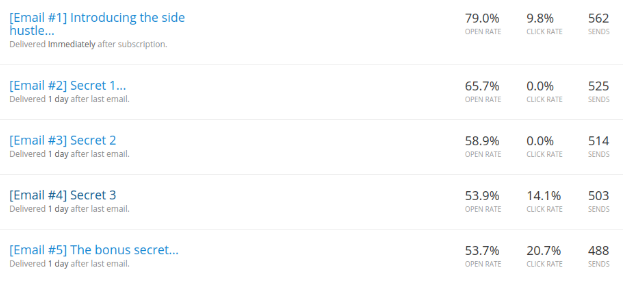This image depicts a computer screen displaying an email sequence within an email marketing application. The screen background is white, and the email list is neatly aligned vertically on the left side. The titles of these emails are highlighted in blue text, while the accompanying information is in black text. 

The sequence starts with "Email number one – Introducing the Side Hustle," which is delivered immediately after subscription. To the right, statistics for the open rate, click rate, and sends are displayed. 

Following this is "Email number two – Secret One," sent one day after the first email. Next is "Email number three – Secret Number Two," also delivered one day after the previous email. The fourth in the sequence is "Email number four – Secret Three," delivered one day after the last email. Finally, "Email number five – The Bonus Secret" is listed, with delivery set for one day after the fourth email. 

Each email title and its details form a straight column from the top-left to the bottom-left of the screen.